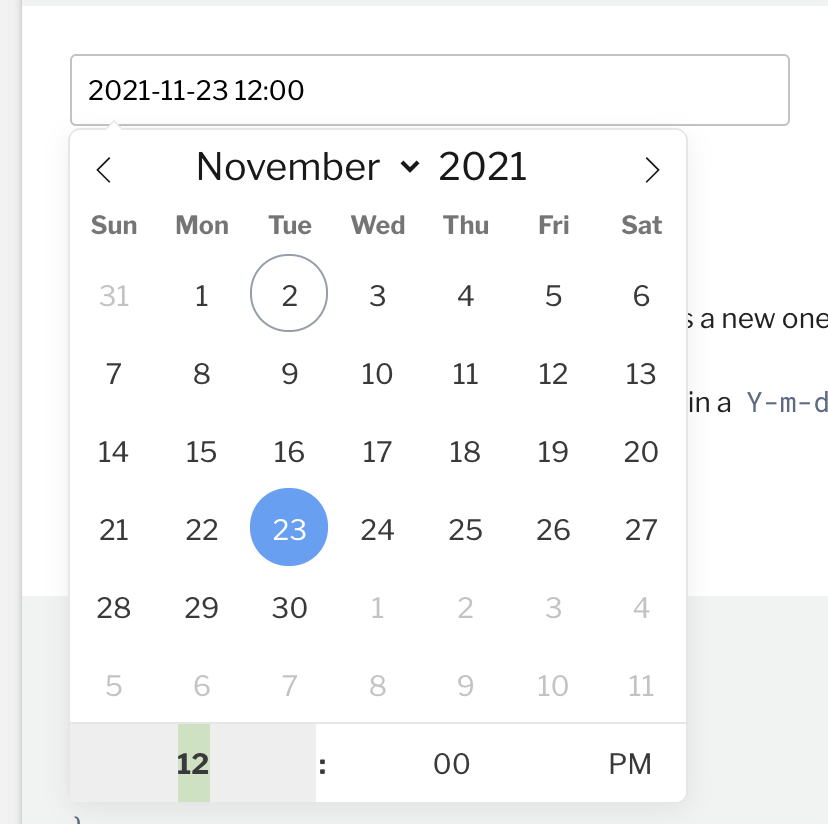The image displays a calendar for November 2021. At the top of the calendar, there is a header bar displaying "2021-11-23" and "12 o'clock." Below this header, the text "November 2021" is prominently featured. The calendar layout starts with Sunday, the 31st of October, and continues through to the 11th of December, ensuring all the dates of November are visible.

Notably, two dates in November are circled: the 2nd is circled in white, and the 23rd is circled in blue with white. Both of these dates fall on a Tuesday, suggesting they are three weeks, or 21 days, apart.

The design of the calendar is primarily minimalist with a white background, black text, and some gray elements. There are slight touches of blue and green. A rectangular, green-grayish section can also be seen, although its function is not clear.

In the background, partially obscured text is visible, with discernible letters and numbers including "A, New, 1, N, A, Y, M, D." The overall composition focuses on the clarity and simplicity of the calendar view, highlighting important dates within the month.